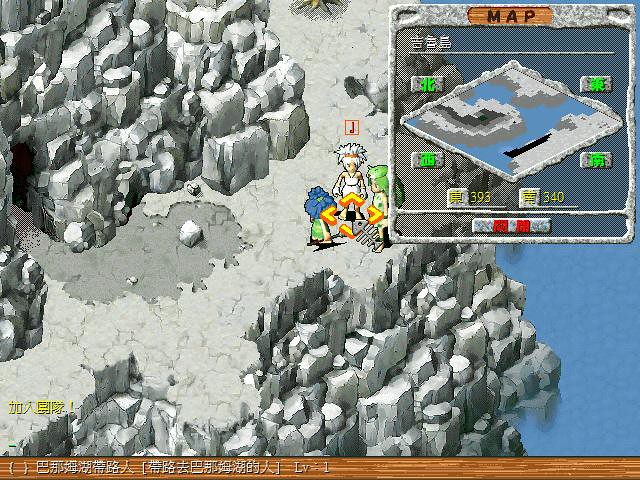The image is a detailed screenshot from a video game, featuring a rocky and mountainous terrain on the left side with a pathway composed of varying shades of gray. On the bottom, a wooden border, light brown and dark brown in alternating pieces, contains black text indicating "LEVEL ONE" in a foreign language. Just above this border, some yellow characters are depicted. To the right, there's a deep blue body of water adjacent to the gray landscape. 

Three characters stand in a circle within the central area. The first character, on the left, is a peach-colored individual with dark blue hair accented by a small lime green dot. They are dressed in a lime green dress with yellow accents. Across from them, two females are visible: one with lime green hair that looks like a creature is perched on her head, wearing a short olive green dress accented with darker green elements, and another with white hair outlined in black. The latter character has a dark brown hairband, an olive-green complexion, white gloves, and a white dress.

A map is situated in the top right corner, showing the landscape in blue and gray colors. The map is enclosed in an orange square with "MAP" written in black letters at the top. Surrounding this map are four labeled buttons, marked in lime green Japanese text. Towards the bottom of the map, points are displayed. 

The floor beneath the characters is a mixture of light and dark gray, strewn with rocks, and sections of a campfire built from light gray and tan logs are visible. Additional details include dark blue water on the right, and the legend accompanying the map shows multiple dark gray squares with splotches of light and mid-gray, containing red and white Japanese text.